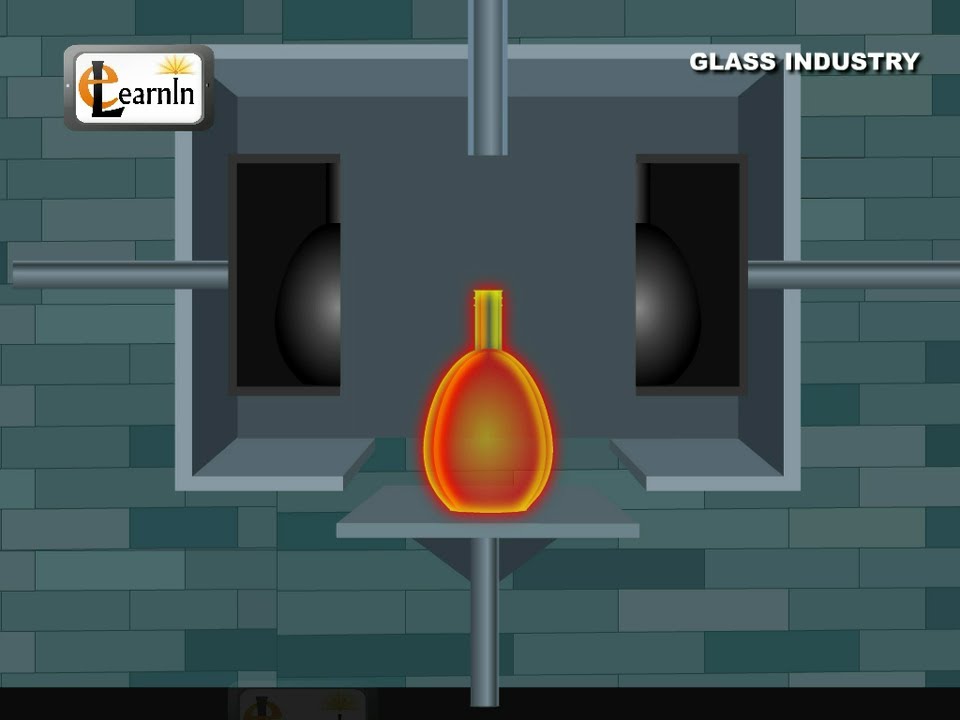The image is a detailed 3D-style drawing designed for online learning about the glass industry, likely from an educational resource called ELEARNIN. It prominently features an illuminated glass bottle, glowing in hues of red-orange with a slightly yellow interior, suggesting it has just been manufactured. The bottle is positioned on a grey steel table, indicative of a glass-making setup. In the background, there is a tealish gray furnace with brick-patterned walls, and rods seemingly directed towards the bottle. The scene has a stylized, cartoonish aesthetic, with a subway tile-patterned wall in greenish-gray hues. Text overlays include "Glass Industry" in the top right corner and "Learn In" stylized as "ElearnIn" in the top left, emphasizing its educational purpose.